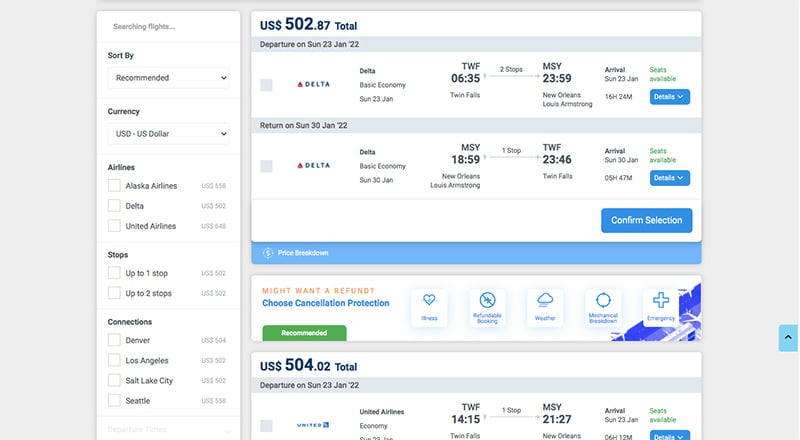This image is a screenshot from a flight booking website showcasing various flight options. On the left-hand side of the interface, there is a white column titled "I'm searching flights," accompanied by several filtering options. These filters include a "Sort By" drop-down menu set to "Recommended," and a "Currency" drop-down menu with "USD - US Dollar" as the first option. There's a section labeled "Airlines" featuring choices like Alaska Airlines, Delta, and United Airlines. Additionally, there are options for layovers, ranging from one to two stops, and listed connection cities including Denver, Los Angeles, Salt Lake City, and Seattle. This section is set against a grayish background.

On the right-hand side, prominently displayed, is a large white box indicating the total price of $502.87 USD. Below this, two different Delta Airlines flight itineraries are detailed. The first itinerary is a departure flight for Sunday, January 23, 2022. This Delta Basic Economy flight departs from TWF (Twin Falls) at 6:35 AM and arrives at MSY (Louis Armstrong New Orleans International Airport) at 11:59 PM, with two stops along the way. The total duration of this flight is 16 hours and 24 minutes. Seats are available, and more details can be accessed.

The second itinerary is the return flight, also with Delta Basic Economy, scheduled for Sunday, January 30, 2022. This flight departs from MSY at 6:59 PM and arrives at TWF at 11:46 PM the same day, with one stop. The total duration for this return trip is 5 hours and 47 minutes. Seats are available, with further details available on selection. There is a confirm selection button at the bottom of this section for finalizing the booking.